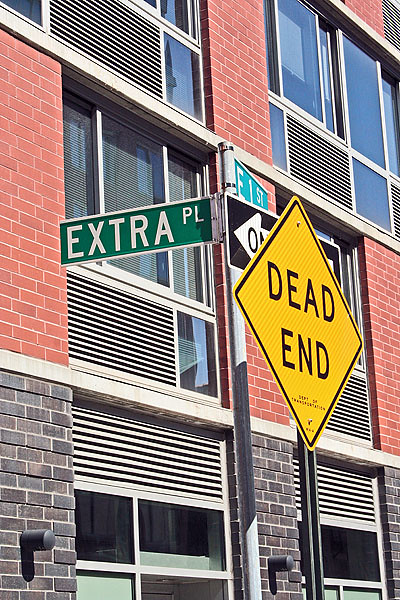The image depicts a street intersection featuring a tall, multi-story brick building as the backdrop. The streets in question are Extra Place and East First Street, marked clearly by street name signs at the corner. At this junction, a 'Dead End' sign is prominently displayed in front of a 'One Way' sign, partially obscuring it; the familiar shape of the 'One Way' sign allows recognition despite the obstruction. The building itself has a base level of gray brick, with the upper stories constructed from standard red brick, extending beyond three visible stories. The scene is brightly illuminated by sunlight, streaming from the top right corner on a clear, sunny day.